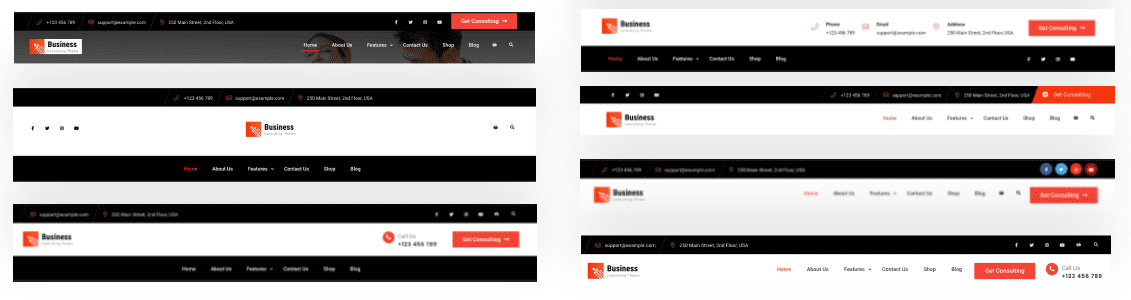The image consists of two distinct screenshots of a business website's interface, showcasing various elements of the site.

In the first screenshot, the website header includes the word "Business" prominently displayed. The top-right corner features navigation links such as Home, About Us, Features, a drop-down for Contact Us, Shop, Blog, and a search function. Additionally, a red "Get Consulting" button is visible along with icons for social media sites like Facebook and Twitter. To the left of these elements, there appears to be an address and contact information. Beneath the header, on the left side, "Business" is displayed within a white-bordered box with some text underneath, accompanied by a red image to its left. Below this section, the address and zip code are centered, followed by a business logo, creating repetitive placement of navigation links such as Home and About Us in a black bar, while the aforementioned elements are reiterated.

In the second screenshot, the layout slightly differs with a more prominent white background compared to black. The business logo is again displayed at the top, along with the phone number, email address, and the red "Get Consulting" button. Below this, the navigation links reappear in a black bar, this time without any underline and in red text. The black bar is visually harmonized with the logo and consulting buttons, which appear in three different instances across the screenshot, mirroring the layout from the first screenshot but with distinct stylistic choices.